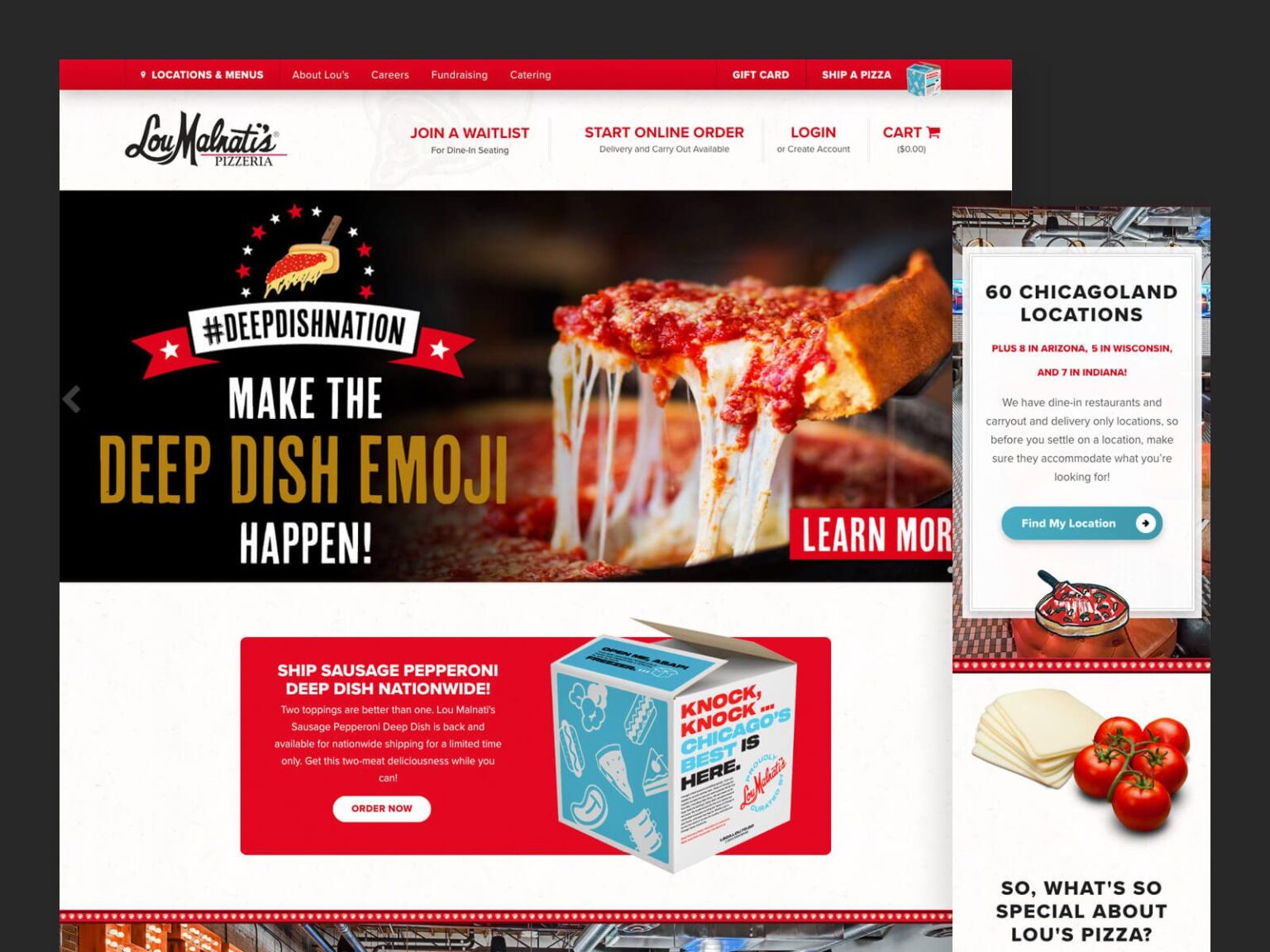In the upper left corner of a long rectangular image, there are the headings "Locations" and "Menus." The name of the establishment, "Lou Malnati's Pizzeria," is prominently displayed in black cursive text. The image features several options: "Join Waitlist," "Start Online Order," "Log In," and a shopping cart icon. The hashtag #DeepDishNation is prominently displayed beside a mouth-watering image of a deep dish pizza. A slice of the pizza is being pulled away, showcasing gooey, melted mozzarella cheese and a rich red sauce atop a thick, golden crust.

Beneath the hashtag, text encourages viewers to "Make the deep dish emoji happen." The caption highlights that Lou Malnati's has 60 locations in Chicagoland, plus additional locations in Arizona, Wisconsin, and seven in Indiana. A blue rectangle labeled "Find My Location" invites users to locate their nearest Lou Malnati's.

An enticing image of sliced cheese and tomatoes accompanies the question, "So what's so special about Lou's pizza?" To the left of this, there is an offer to "Ship sausage pepperoni deep dish nationwide." A blue box on the side reads, "Knock, knock! Chicago's Best is Here," with an option to "Order Now."